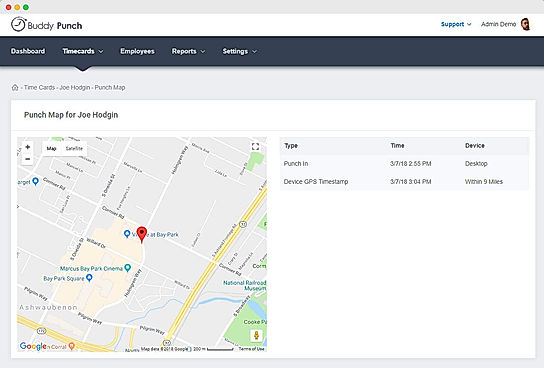The image showcases a website interface designed for monitoring employee time punches via a map. At the top of the screen are red, yellow, and green indicators reminiscent of those found on Apple computers, indicating window controls. In the upper left corner is the "Buddy Punch" logo. Just beneath this, a blue rectangular banner spans the width of the screen, featuring navigation options labeled "Dashboard," "Time Cards," "Employees," "Reports," and "Settings." Below the banner, the text reads "Time Cards," "Joe Hodgin," and "Punch Map," suggesting a focus on tracking Joe Hodgin's punched-in locations. The map on the website displays various locations where employees presumably clock in and out. The area on the map is labeled "Ash Wildbanon," a location unfamiliar to the observer.